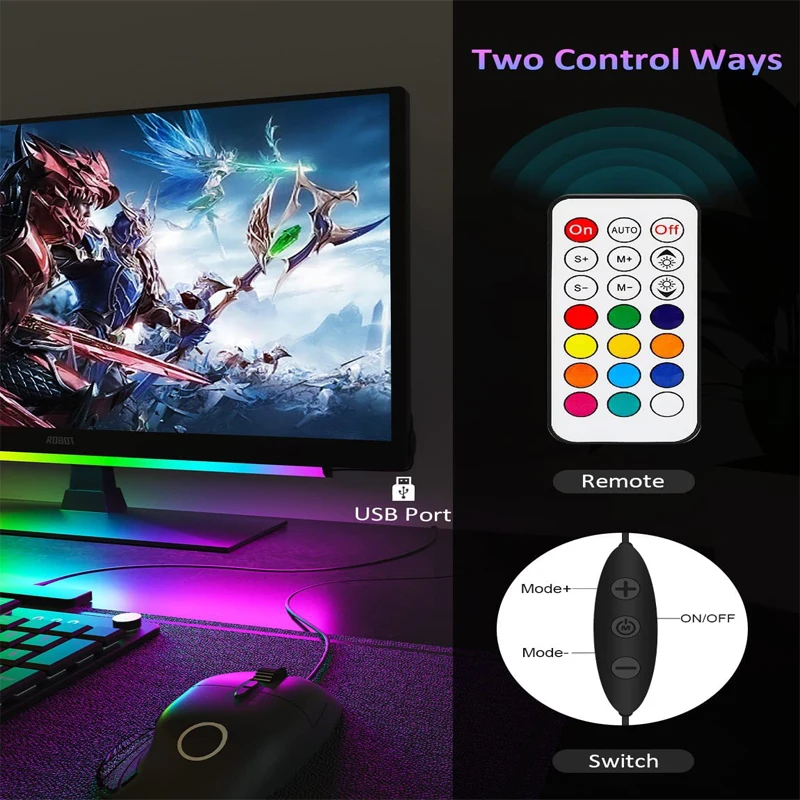The image depicts a detailed setup for a computer gaming system, centered around a large monitor on the left side of the screen that displays a mythical combat scene. The monitor has the word "robot" at the bottom, with connected RGB lighting featuring all colors. The screen showcases creatures clad in colorful armor, including a flying creature with blue wings wielding a large blue bow and arrow. Below the monitor is a sleek black desk, equipped with a wired keyboard and mouse. The cords for these devices trail underneath the desk towards the back wall. Near the left bottom corner of the monitor, a "USB port" is indicated by white text and a USB symbol.

To the right of the image is a detailed depiction of a remote control, described in advertising material. At the top of the remote, in a purple-to-pink gradient, bold text reads "two control ways." The remote features various buttons with color-coded functions: red for "on," white for "auto," and options for controlling the RGB lights and modes. Central buttons include an up-arrow-over-sun icon, down-arrow-over-sun icon, and several color-coded buttons: red, green, purple, yellow, orange, blue, pink, and green with a corresponding "M" and "S" marked with "+" and "-" signs. Below these buttons is the word "remote." Another section of the remote highlights additional controls like "mode plus," "mode minus," "on," "off," and "switch."

A black strip with white background highlights the remote control’s functions and RGB settings in an organized manner, creating a comprehensive and colorful portrayal of the entire system.